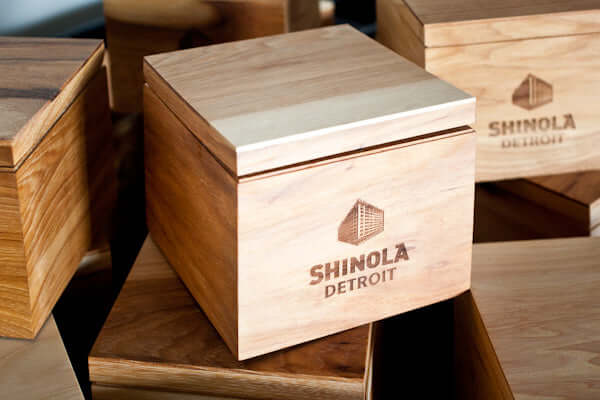The image showcases a collection of approximately nine or ten carved wooden boxes with lids, predominantly in shades of tan and light brown. These boxes, stacked and scattered across the frame, almost fill the entire image, suggesting a warehouse or storage environment. Each box features prominently displayed logos with the text "Shinola, Detroit," and an image of a square building printed on the front. One box, positioned diagonally in the front, stands out among the unevenly placed others. The scene also includes a mysterious object in the top left corner that remains indistinct. The overall setting hints at an area storing an excess amount of this particular product.